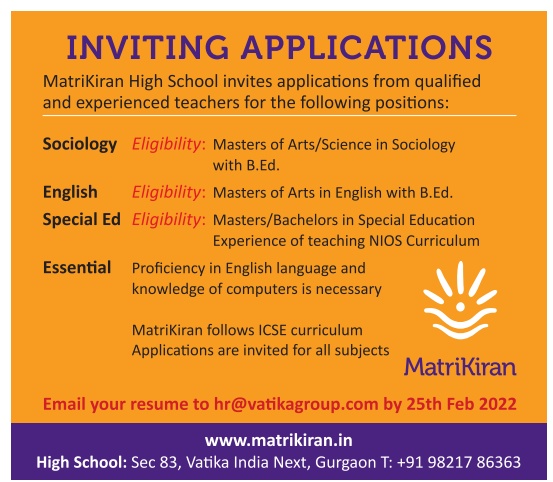This image appears to be a cropped screenshot from a tablet or desktop, where the web address, browser, and operating system are not visible. At the top, in large purple capital text, the headline reads "Inviting Applications." 

Below, in black text, the announcement states that "Matrikiran High School invites applications from qualified and experienced teachers for the following positions." The positions listed include:

- **Sociology**: Eligibility criteria in red text specify a Master of Arts/Science in Sociology with a B.Ed.
- **English**: Eligibility criteria state a Master of Arts in English with a B.Ed.
- **Special Education**: Eligibility criteria state a Master's or Bachelor's in Special Education, with experience in teaching an IOS Curriculum essential. 

Additionally, the post mentions the necessity for proficiency in the English language and computer knowledge. It clarifies that Matrikiran High School follows the ICSE curriculum and applications are invited for all subjects.

The name "Matrikiran" is mentioned again in purple near the bottom, followed by a white icon resembling an eyeball with the sun. In red print, it instructs applicants to email their resumes to hr@vatikagroup.com by February 25, 2022. The school's website, www.matrikiran.in, is listed, along with the high school's location: Sector 83, Vatika, India, and Gurgaon, spelled as "Gurgaon." The contact telephone number provided is +919821786363. The school is actively seeking qualified teachers to join its faculty.